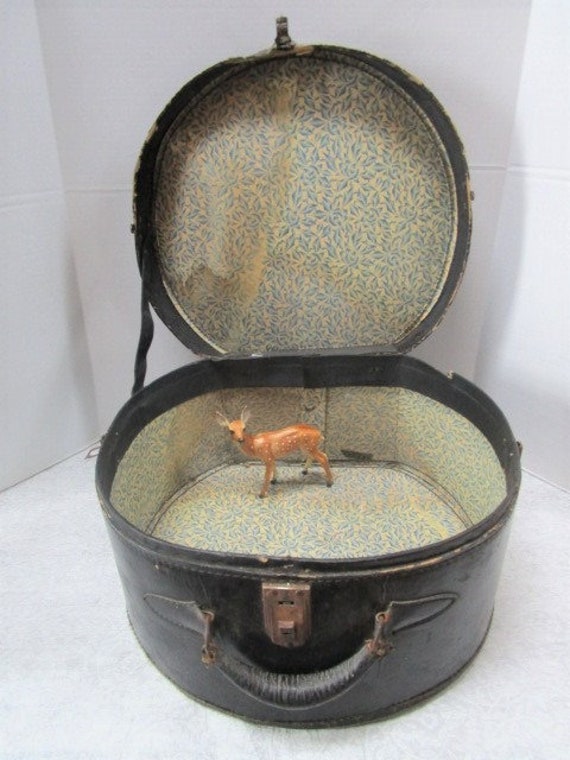The image is a detailed photograph of a small toy deer, resembling Bambi, placed inside a weathered, black leather hatbox. The hatbox is round and resembles an old clutch bag or carrying case. The exterior is black leather, showing signs of wear and tear, with a leather-wrapped curved handle featuring a rusted clasp and latch. A hinge and a strap on the side limit the lid's opening. 

Inside, the hatbox is lined with an off-white background adorned with blue flower or leaf patterns. The lining extends to the inside of both the lid and the bottom, where a visible staple and stitching outline the edges. A plastic gear is noted in the bottom corner.

The toy deer is brown with white spots, indicative of a doe as it has no antlers. The hatbox and toy deer are positioned against a white or slightly bluish-white backdrop, possibly paper, under good lighting that suggests a professional setting like an eBay listing.